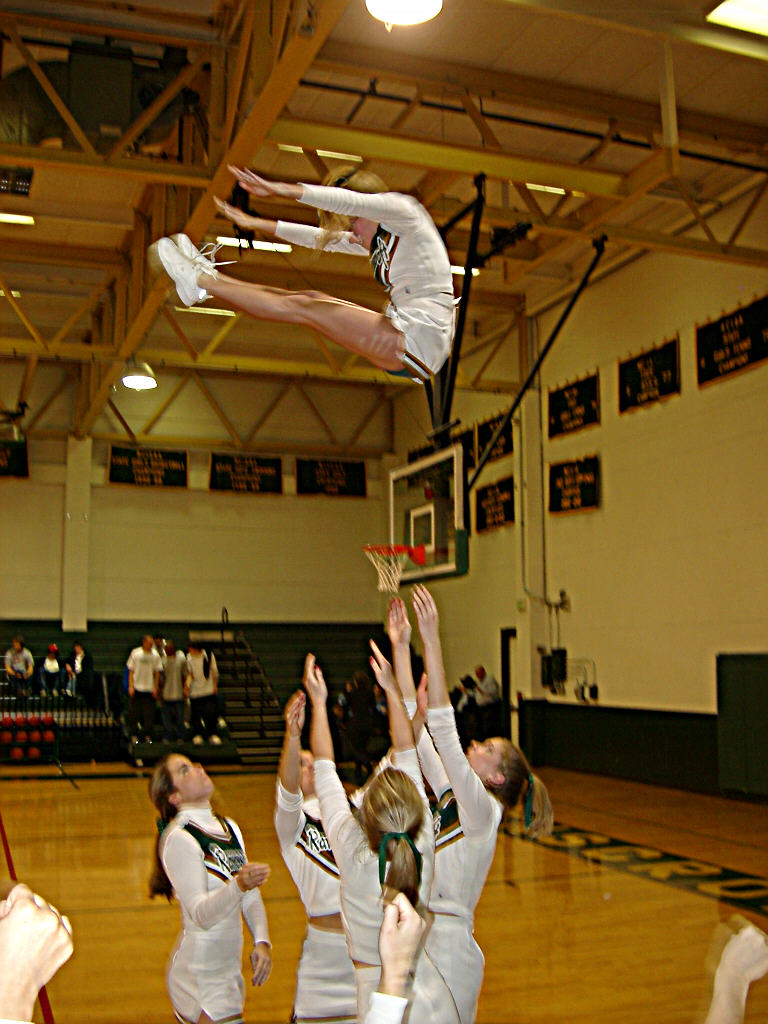In this vibrant photograph taken inside a gymnasium, the focal point is a dynamic scene of cheerleaders performing or practicing their routine. Dominating the image is a basketball hoop mounted from the ceiling, complete with a white net and a red metal ring, set against a backboard. Below the hoop, several cheerleaders are positioned closer to the camera. They are donned in uniforms that predominantly feature white, embellished with patterns of black and maroon, while their hair is neatly tied back with green ribbons.

A standout element in the image is a cheerleader launched high into the air. Captured mid-motion, her body forms an arch with her arms and legs extended forward, almost reaching for her toes. She sports white sneakers and a matching uniform, while her blonde hair flows from a high ponytail. The camera has caught her in a side profile from her shoulder down, highlighting the movements and strains of her routine.

The gymnasium's interior is well-illuminated, revealing an exposed beam ceiling painted light yellow with visible steel and wooden structures. The backdrop features several rectangular banners in black with orange writing, celebrating the team's victories. Blue posters with yellow accents line the walls, adding to the vibrant atmosphere. Bleachers along the far side host a few spectators, whose presence contributes to the lively setting. The intricate details, from the cheerleader’s pose and outfit to the gymnasium’s structural and decorative elements, collectively encapsulate the energetic essence of this moment.